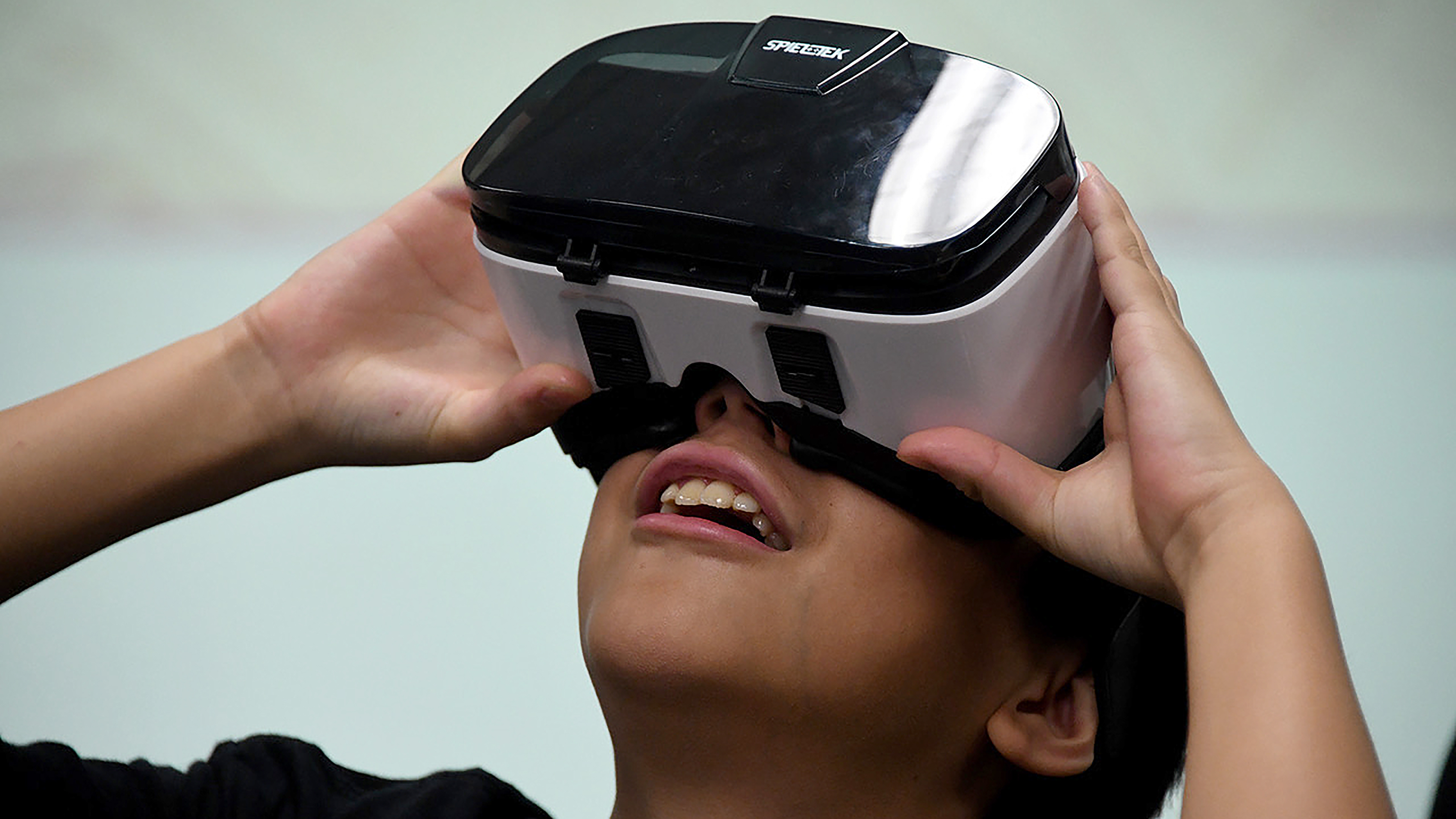The photograph captures a young boy, around 10 to 12 years old, intensely engaged with a virtual reality (VR) headset. The boy, with short dark hair and dark skin, is looking up and to the left with his mouth slightly open, conveying a sense of awe or curiosity. The VR headset, which consumes the entire upper part of his face, is predominantly black with white sides and features white lettering on the top that reads "SPIELTEK". The lower part of the device, including the eye pads and nose straps, is black, closely fitting his face. The child is holding the VR headset firmly with both hands, wearing what appears to be a black shirt, although only the top of it is visible. The background is a very blurry light bluish-gray, creating a soft contrast that emphasizes the boy and his VR headset. In the bottom right corner, a small sliver of black slightly intrudes into the frame, possibly hinting at another person or object, though it remains indistinct.